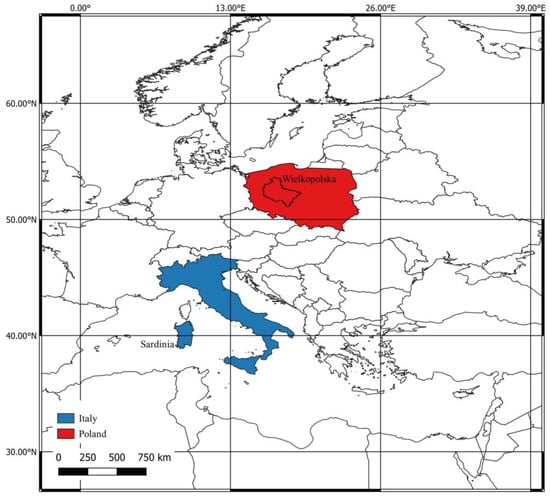This image depicts a detailed black-and-white map of Europe accented by red and blue colorations for specific countries. The map features a grid of longitudinal and latitudinal coordinates, with east coordinates ranging from 0 to 39 degrees and north coordinates from 30 to 60 degrees. Poland is highlighted in red and labeled as "Wielka Polska," while Italy, including Sardinia and Sicily, is shaded in solid blue. Other European countries are outlined in black. A small key on the left side indicates the color codings for Poland and Italy, alongside a black-and-white measurement bar showing distances from 0 to 750 kilometers.